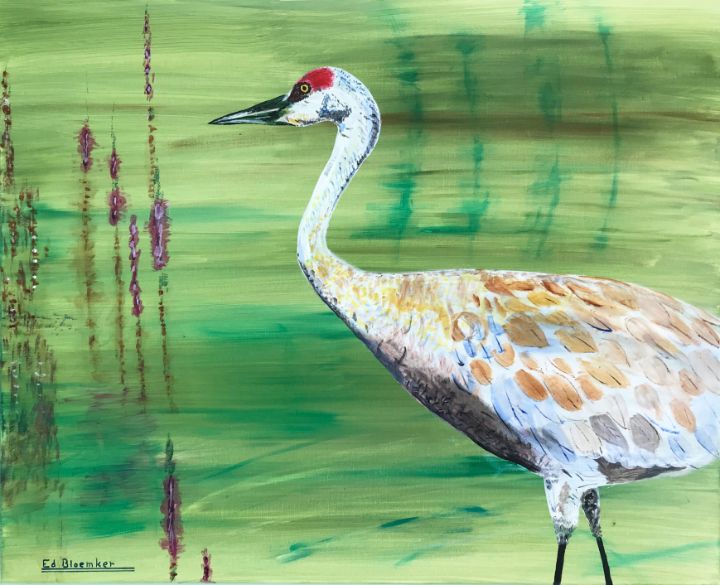In this detailed painting by Ed Blomker, prominently signed in the lower left corner with two underlines beneath his name, an elegant bird, likely a heron, takes center stage against a nuanced background. The scene is set in a shallow, pond-like environment faithfully represented through a harmonious mix of light green and darker green streaks, evoking gentle water ripples or grass. On the left side, purple flowers, perhaps lavender or a similar water plant, rise from the water, adding a touch of vivid color to the composition.

The bird itself, facing left, showcases delicate features with its spindly black legs and a curved neck that culminates in a long, dark pointed beak. Its plumage is primarily white, highlighted with brown, beige, light blue, and golden patches that texture its back and wings. Adding to its detailed appearance, the heron sports striking red markings above its gold-hued eye, with additional gray and tan accents seamlessly blending into its overall feather design. The bird's imposing yet graceful stature, merged with the lush and tranquil setting, brings a sense of realism and serenity to the artwork.